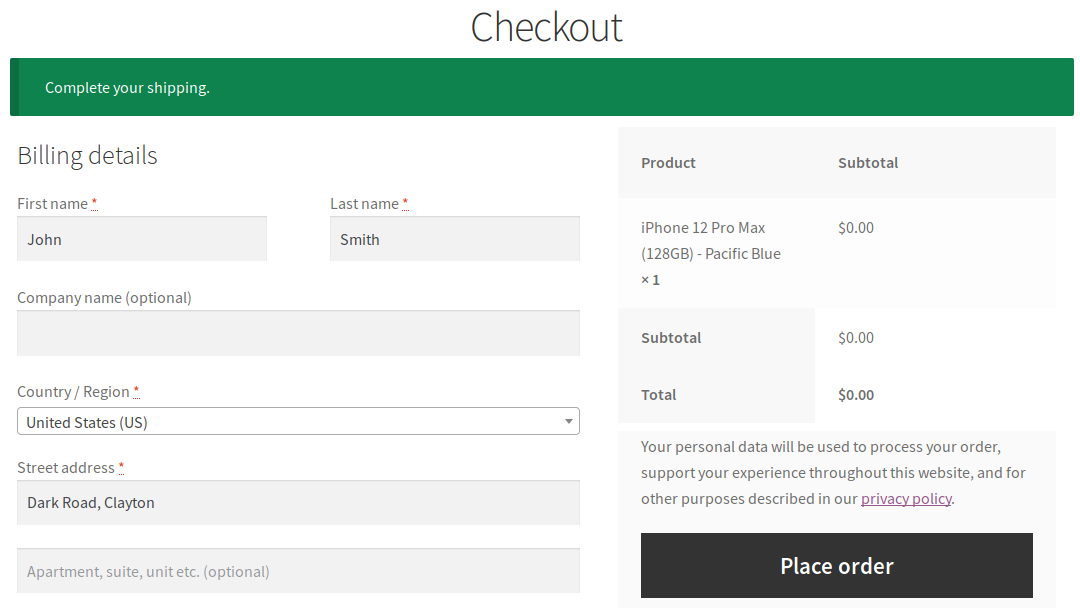This is a detailed screenshot of a checkout page. At the top, there is a header that reads, "Checkout." Beneath it, there is a green banner with small white text that says, "Complete Your Shipping."

Below the banner are sections for billing details with multiple fields. The first line contains fields for "First Name" and "Last Name," which are filled in with "John Smith." The next line has an optional field for "Company Name," which is empty. Following that, the field for "Country/Region" shows "United States (US)." The "Street Address" field contains "Dark Road, Clayton," and there is an additional field for "Apartment, Suite, Unit, etc. (optional)," which is also empty.

On the right-hand side of the page, there are two columns labeled "Product" and "Subtotal." Listed under "Product" is "iPhone 12 Pro Max 128GB in Pacific Blue," with a quantity of one. The subtotal is "$0.00," making the total also "$0.00."

At the bottom, there is a note stating that personal data will be used to process the order, support the user's experience throughout the website, and for other purposes as described in the privacy policy.

Finally, there is a large black button with white text that says, "Place Order."